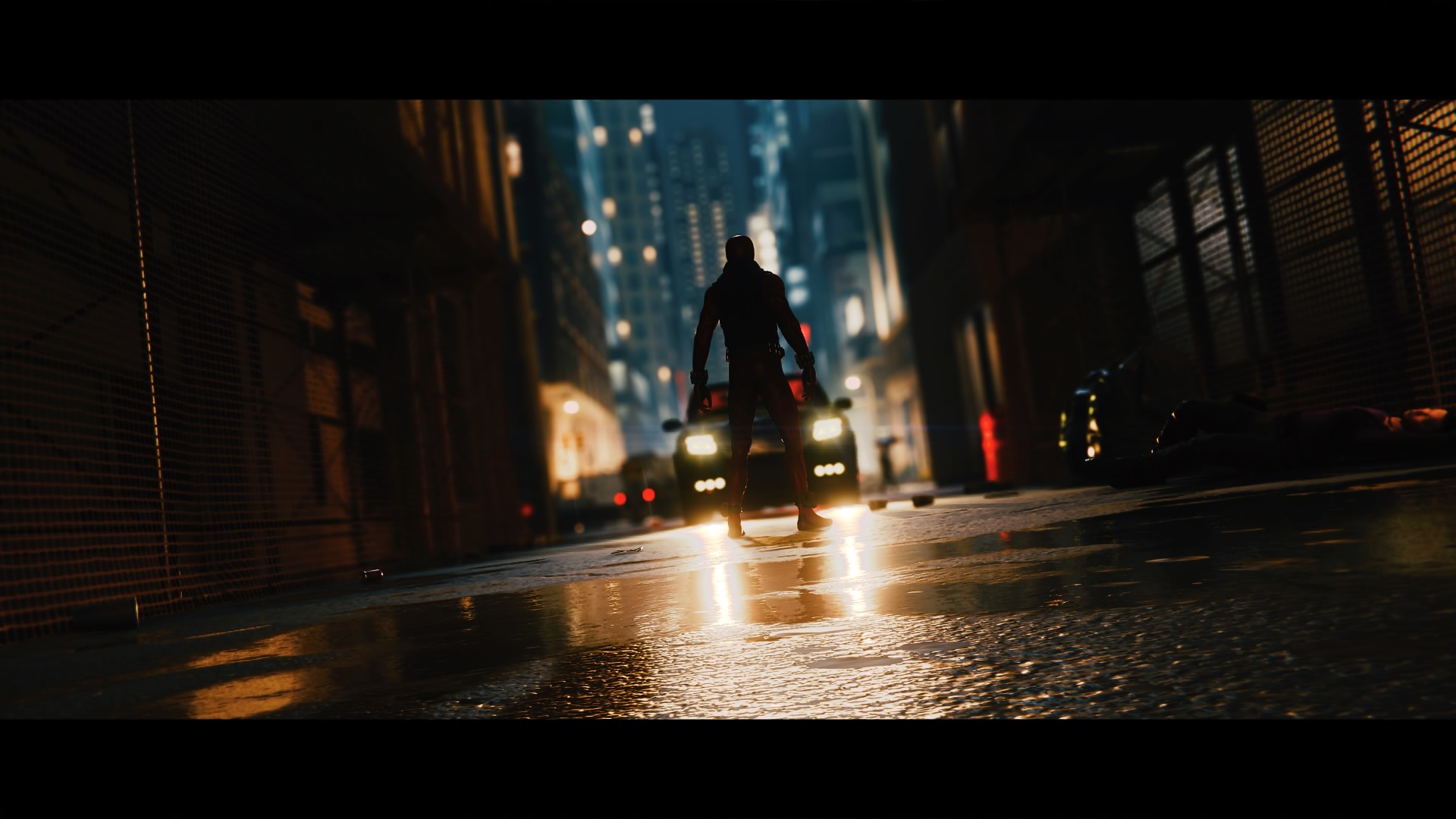A dark, desolate street is captured in this atmospheric nighttime scene. The wet asphalt glistens under the reflection of the car's headlights, creating a sharp contrast against the black surface. A car is driving towards the camera, its bright lights piercing through the night. Standing in its path is a lone figure, possibly dressed in a suit and an overcoat, adding an air of mystery. A large puddle of water is visible on the road, contributing to the reflective surfaces. On the left side of the image, there's a building, while on the right, a closed gate with black bars stands prominently. In the far background, a sprawling cityscape with tall, high-rise buildings, many windows aglow, stretches upwards. Various kinds of lights illuminate parts of the scene, and to the right of the car, a lit sign adds another layer of human presence to the urban night.